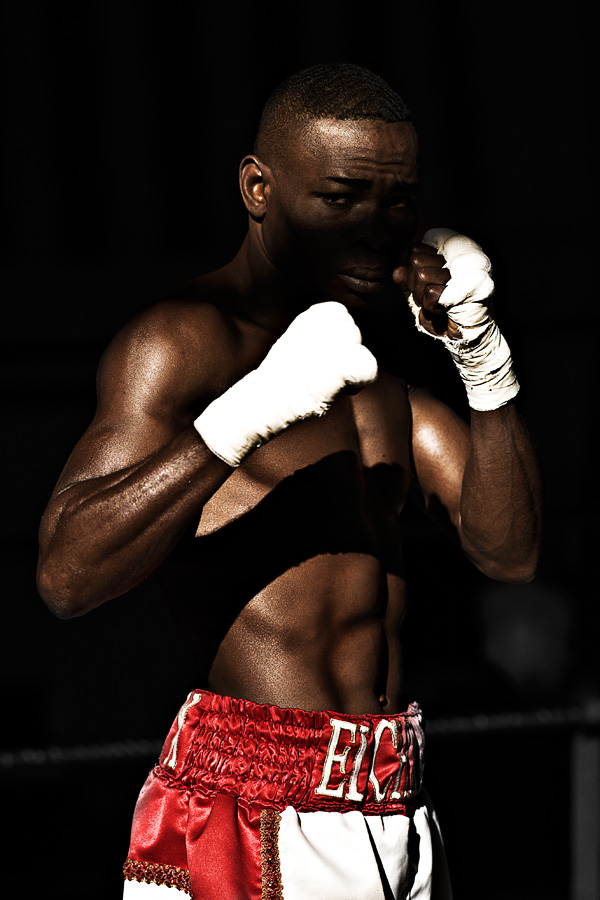The image portrays a highly toned boxer in a ready-to-spar stance, facing the viewer with his arms upraised in a defensive position. The boxer, a black man with very short dark hair, is shirtless and clad in white and red shorts that exhibit partially visible lettering. His fists and wrists are wrapped in white protective cloth. The scene is bathed in dramatic lighting, casting deep shadows on his nose and cheek areas, and starkly illuminating his muscular physique. There's a noticeable glare from the left side, emphasizing the shadows cast across his midsection by his upraised arm. The setting appears to be a boxing ring, suggested by the faint, out-of-focus rope visible near the bottom of the image. The background fades to solid black above his elbows, intensifying the contrast and adding to the artistic quality of the photograph.